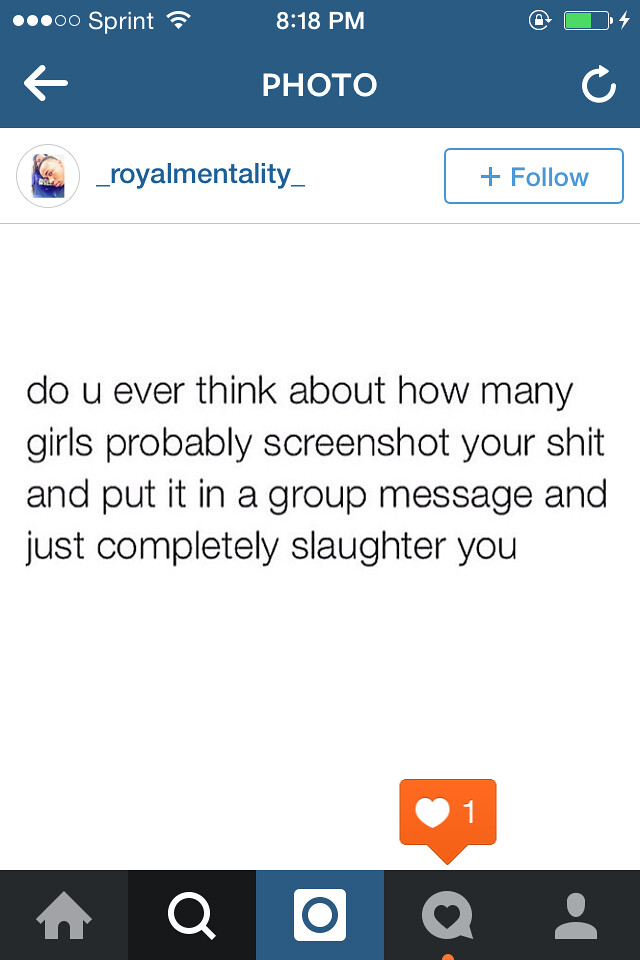The image is a screenshot from a smartphone displaying the Instagram feed of Royal Mentality. The screen captures a quote in all lowercase, which reads: "do you ever think about how many girls probably screenshot your shit and put it in a group message and just completely slaughter you?" The background of the image includes standard user interface elements: at the top, it shows that the phone carrier is Sprint, the time is 8:18 p.m., the battery is about 70% charged, and Wi-Fi is enabled. The bottom of the screen features icons for the homepage, search, social media, notifications, and user profile. The post by Royal Mentality, adorned with a single heart icon indicating one like, suggests a level of resonance with at least one viewer amidst its provocative and candid tone.